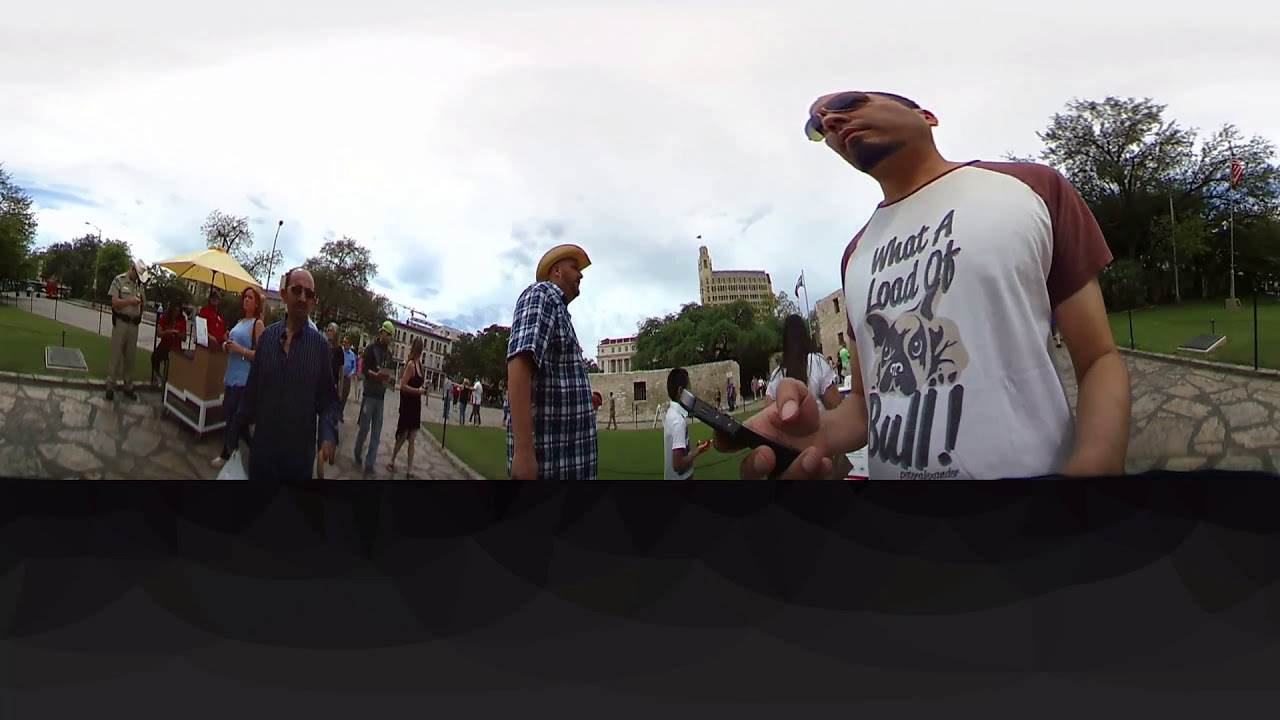In a bustling city park surrounded by low-rise buildings, a diverse crowd of over 20 people is captured in motion, participating in what seems to be a community event. The scene is dominated by a man in the foreground wearing oval-shaped, brown-tinted sunglasses and a quirky shirt that reads, "What a load of dog poo," accompanied by an image of a pitbull resting its head on its legs. He holds a black phone in his right hand while his left remains out of view. To his left, a man in a cowboy hat and checkered shirt stands out, and nearby, another man sports a blue shirt. Further back, a security guard is stationed near a food court adorned with a yellow umbrella. The park's stone pathways are lined with grass on either side, adding a touch of greenery. Despite the cloudy sky with occasional patches of blue, the atmosphere is lively as people mill about, some near a stand that appears to be either selling food or distributing brochures.